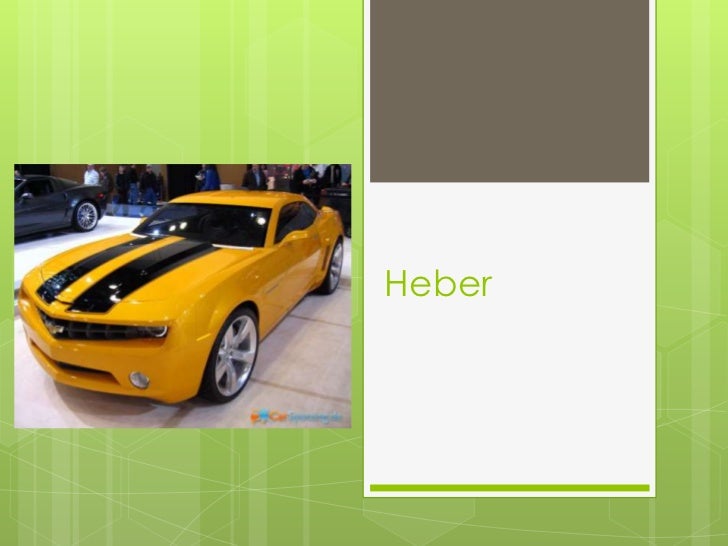The image resembles an unfinished presentation slide with a bright green background featuring vertical stripes and faint, curved lines. On the left side, a photograph of a shiny, deep yellow (possibly light orange) sports car, likely a Mustang but perhaps a Chevy Camaro, prominently captures attention. The car boasts two black stripes running down its hood, a hood scoop, and chrome or silver-spoked wheels. Behind the car, curious observers are visible, indicating it's probably displayed in a showroom. Adjacent to the car's photo, on the right side of the slide, is a large white rectangle topped with a gray area. At the bottom, the word "Heber" is written in lime green text.